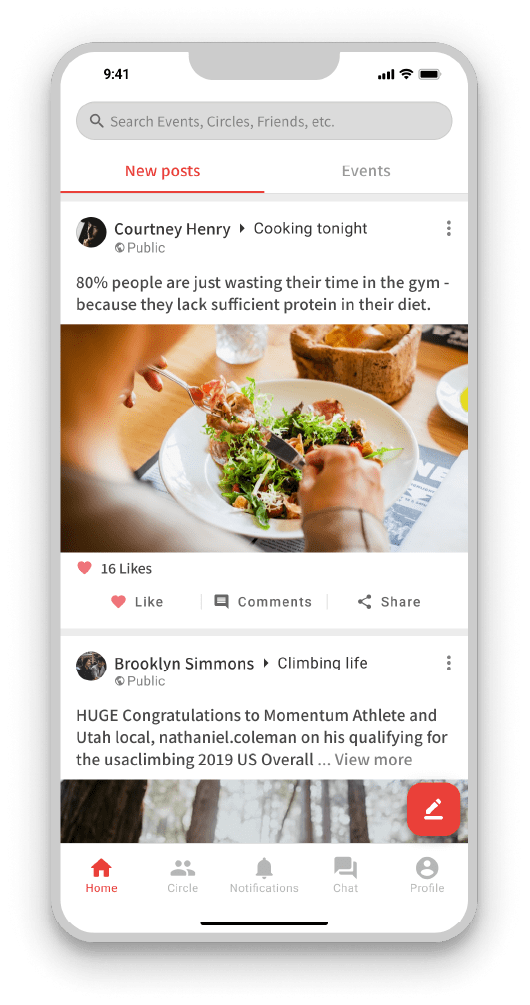The screenshot from a smartphone displays a social media app interface at 9:41 AM. At the top, a search bar is prominently available for easy navigation. Below, two tabs are visible: "New Post," highlighted in red with an underlining, and "Events," displayed in gray. The highlighted "New Post" reveals Courtney Henry's contribution to the "Cooking Tonight" group, stating, "80% of people are just wasting their time in the gym because they lack sufficient protein in their diet." Accompanying this post is an image of a woman enjoying a salad, possibly at a restaurant or at home, indicated by the presence of a tablecloth or placemat. The woman is using a fork and knife, and the post has garnered 16 likes, with options to comment and share. Below this post, Brooklyn Simmons from the "Climbing Life" group congratulates Momentum athlete and Utah local Nathaniel Coleman for qualifying for the USA Climbing 2019 U.S. Overall competition, with an option to "view more" details.